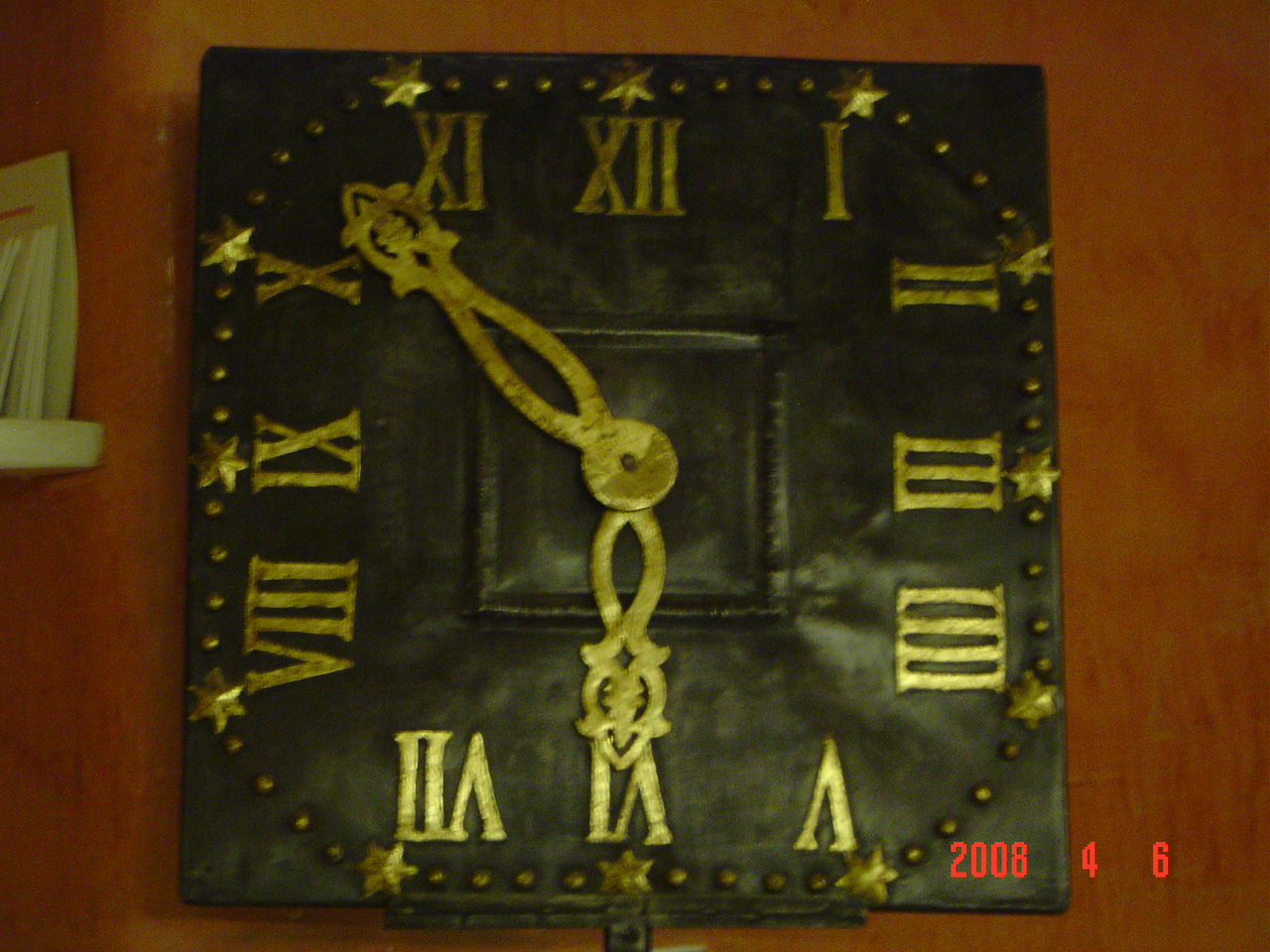This image showcases an artistic and antique clock mounted on a wooden wall, with a small shelf to the left holding folded papers or mail. The clock features a square design with a mostly black face, adorned with golden Roman numerals from I to XII. The hour hand points to VI, while the minute hand is positioned between X and XI. Both clock hands are intricately designed with elegant, fancy shapes reminiscent of letter openers. The clock's face includes golden dots and stars along the edges, creating a visually striking pattern. Notably, the bottom right of the clock face displays the inscription "2008, 4, 6."